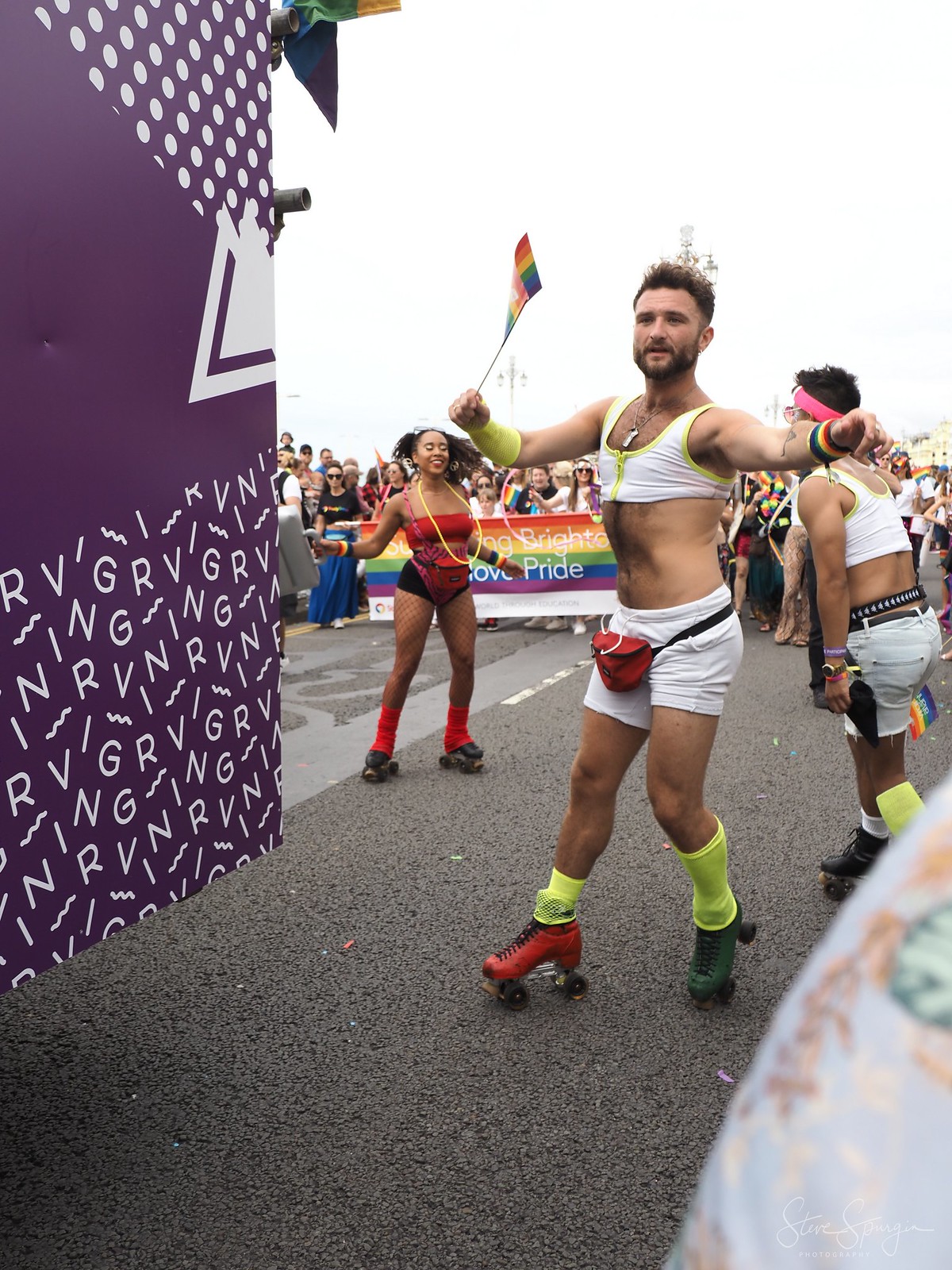The photograph captures the vibrant beginning of a gay pride parade on an overcast day. In the foreground, three individuals on roller skates are prominently featured. The central figure, a man, is wearing a white sleeveless cutoff shirt that reveals his chest, white shorts, yellow socks, red and black roller skates, and a red fanny pack. He holds a raised gay pride flag in his right hand. To his left stands another man, similarly dressed in white shorts and a white sports bra, with a red headband and a belt around his waist. On the right is a black woman wearing a red top and brown shorts, accessorized with yellow beads around her neck. She wears red and brown jersey roller skates and holds a flag. In the background, a large rainbow-colored banner with the words "Love Pride" is carried by a group of people marching forward. To the far left, a purple billboard with the letters "GRV" in white letters can be seen. The scene is bustling with participants demonstrating their pride and solidarity.